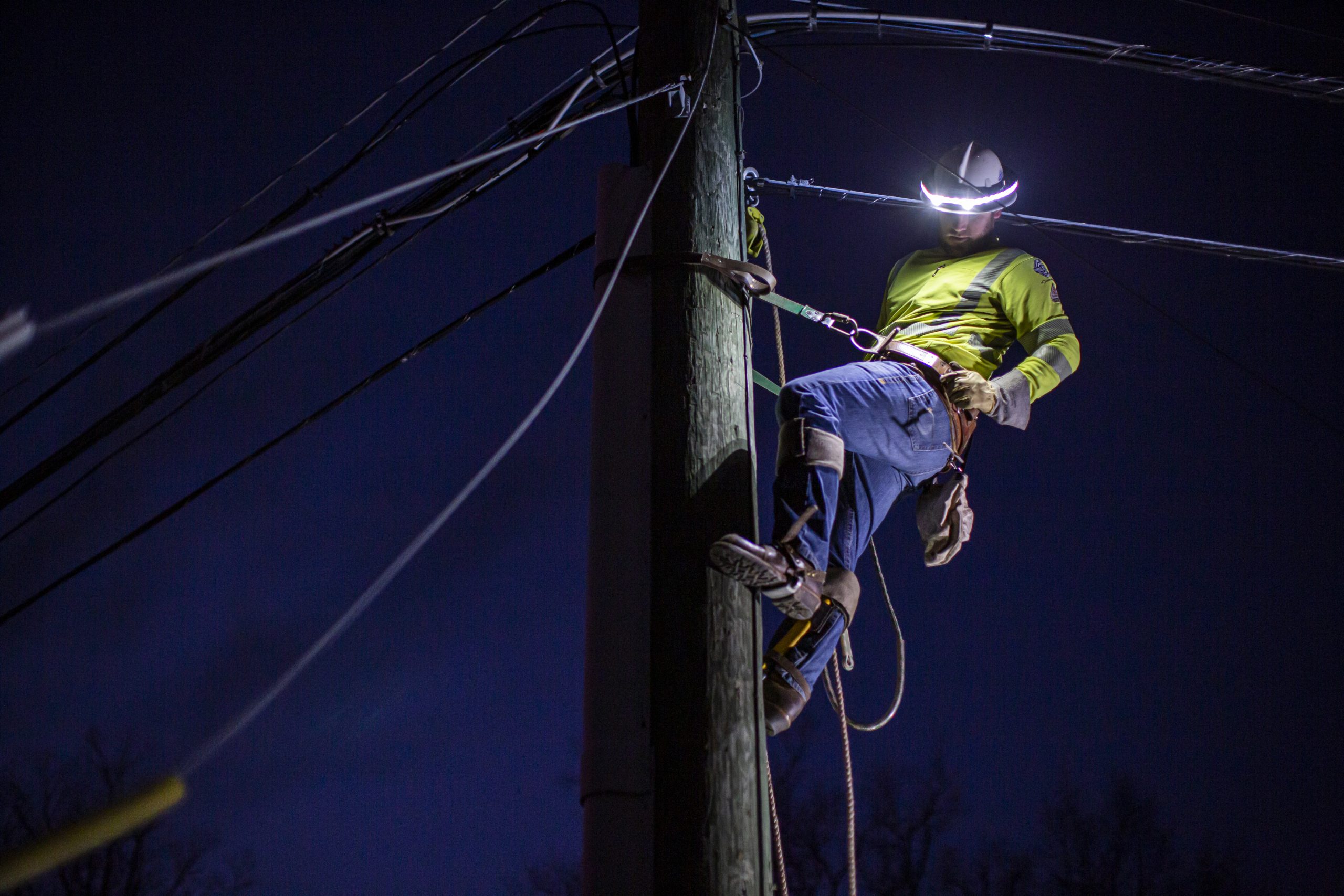In this nighttime photograph, a lineman is diligently working atop a wooden utility pole under a dark, star-speckled sky. Clad in a bright yellow shirt and blue jeans, he is securely attached to the pole with a waist belt that loops around it and climbing spikes fastened to his work shoes. His hard hat, equipped with a light, illuminates his work area as he reaches into his tool belt, likely retrieving the necessary tools for his task. This dedicated worker, positioned on the right side of the image, is surrounded by a network of electrical or phone lines extending outward from the pole, with some wires loosely hanging to the left, possibly indicating the focus of his repair. The scene also features silhouettes of leafless trees at the bottom, adding a touch of nature to this industrious nighttime endeavor.